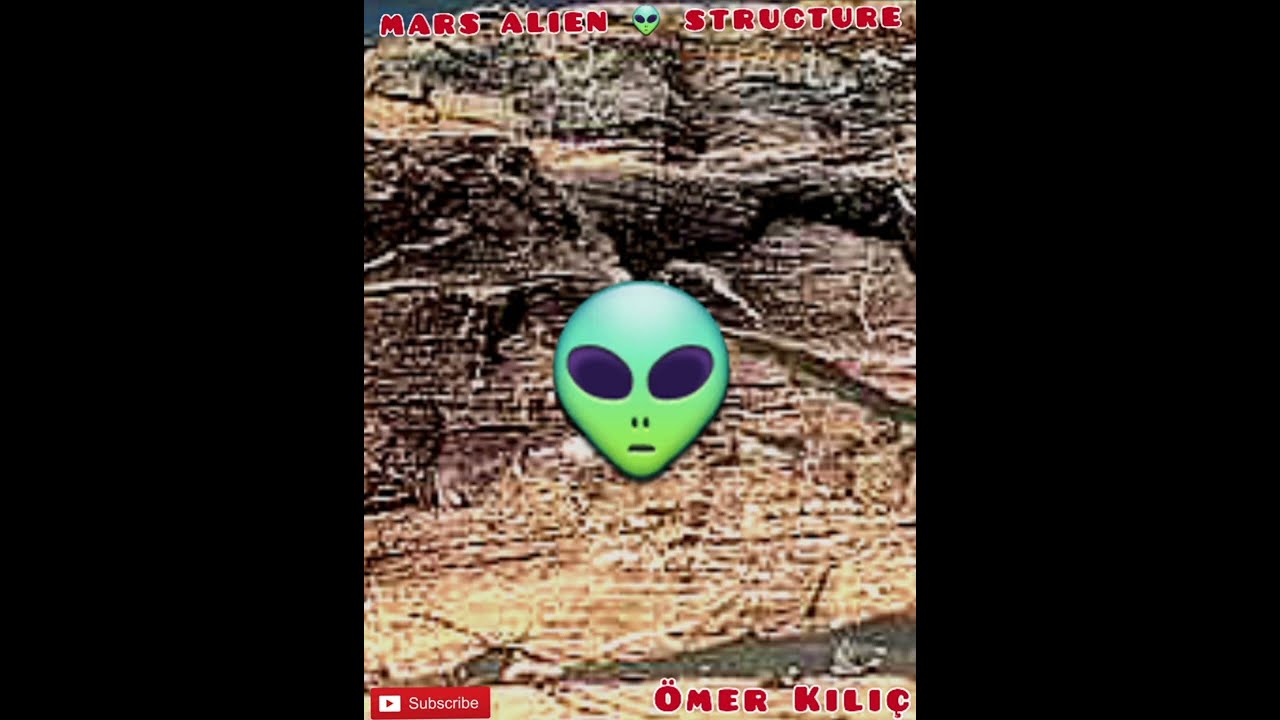The image features a portrait-oriented, pixelated photograph of a rocky canyon, possibly resembling the Grand Canyon, with jagged, brownish rock formations. In the center, there is a striking clipart image of a green alien head with large, black, oval eyes pointed inward, two nostrils, and a simple, straight line for a mouth. At the top of the image, bold red letters with white outlines spell out "MARS ALIEN," with an additional small alien head emoji beside it. Immediately below, the text continues with the word "STRUCTURE." The bottom left corner showcases a YouTube subscription prompt with a red box and white font saying "subscribe" accompanied by an arrow. In the bottom right corner, the name "Omer Kılıç" appears in red letters with a white outline. Black vertical bands frame the left and right edges of the image.